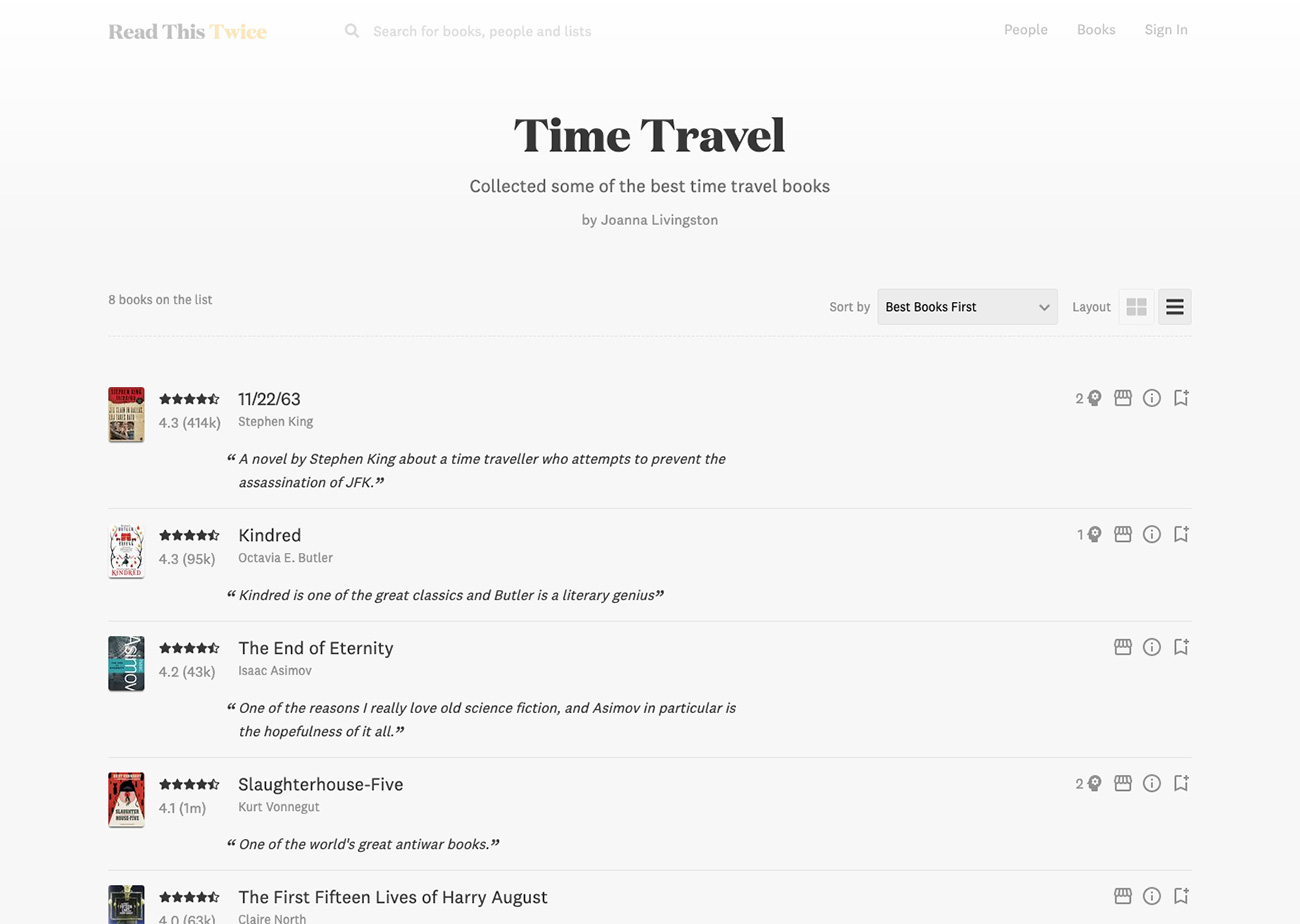This image showcases a book recommendation website with a focus on time travel literature. The interface features a predominantly white background with black text. At the top, a drop-down menu allows users to sort books by categories, with the current selection set to "Best Books First." Users can also toggle the layout between list and picture views, with the list view currently displayed. 

The top-rated book is "11/22/63" by Stephen King, earning a 4.3-star rating. A thumbnail of the book cover shows a red top with a white banner. The brief description reveals it is a novel about a time traveler attempting to prevent JFK's assassination. 

Following that is "Kindred" by Octavia E. Butler, also rated 4.3 stars. The synopsis highlights its status as a classic and praises Butler's literary craftsmanship. 

Next is Isaac Asimov’s "The End of Eternity" with a 4.2-star rating. A quoted review emphasizes the hopeful nature of science fiction, particularly Asimov's works, as a standout aspect. 

Kurt Vonnegut’s "Slaughterhouse-Five" follows, rated at 4.1 stars, and recognized as one of the great anti-war books. 

Finally, "The First Fifteen Lives of Harry August" by Claire North is listed with a 4-star rating. 

A series of symbols appears on the left-hand side of the screen, though their significance is unclear.